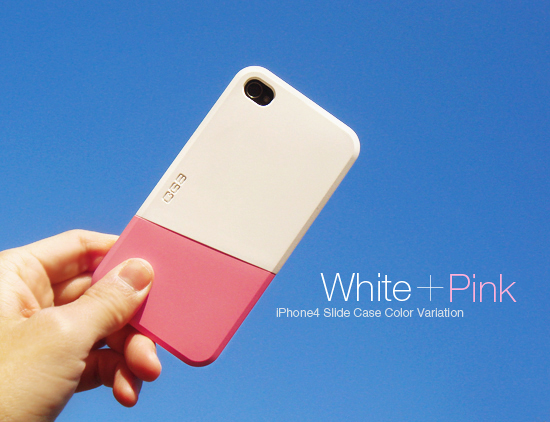The advertisement features a phone case for the iPhone 4 against a clear blue sky background. On the left side of the image, a hand holds the phone case, tilting slightly to the right. The case itself is stylishly divided into two sections, with the upper third in white and the lower two-thirds in pink, reminiscent of classic pink and white erasers. Only the thumb and lower fingers of the hand are visible as they grip the phone, with the camera peeking out from the top left corner of the case. To the right, white text reads "white plus," followed by the word "pink" in pink font. Below this is more white text that states, "iPhone 4 slide case color variant," suggesting the ability to switch or slide the case. The overall design emphasizes the color variation and modern aesthetic of the product.